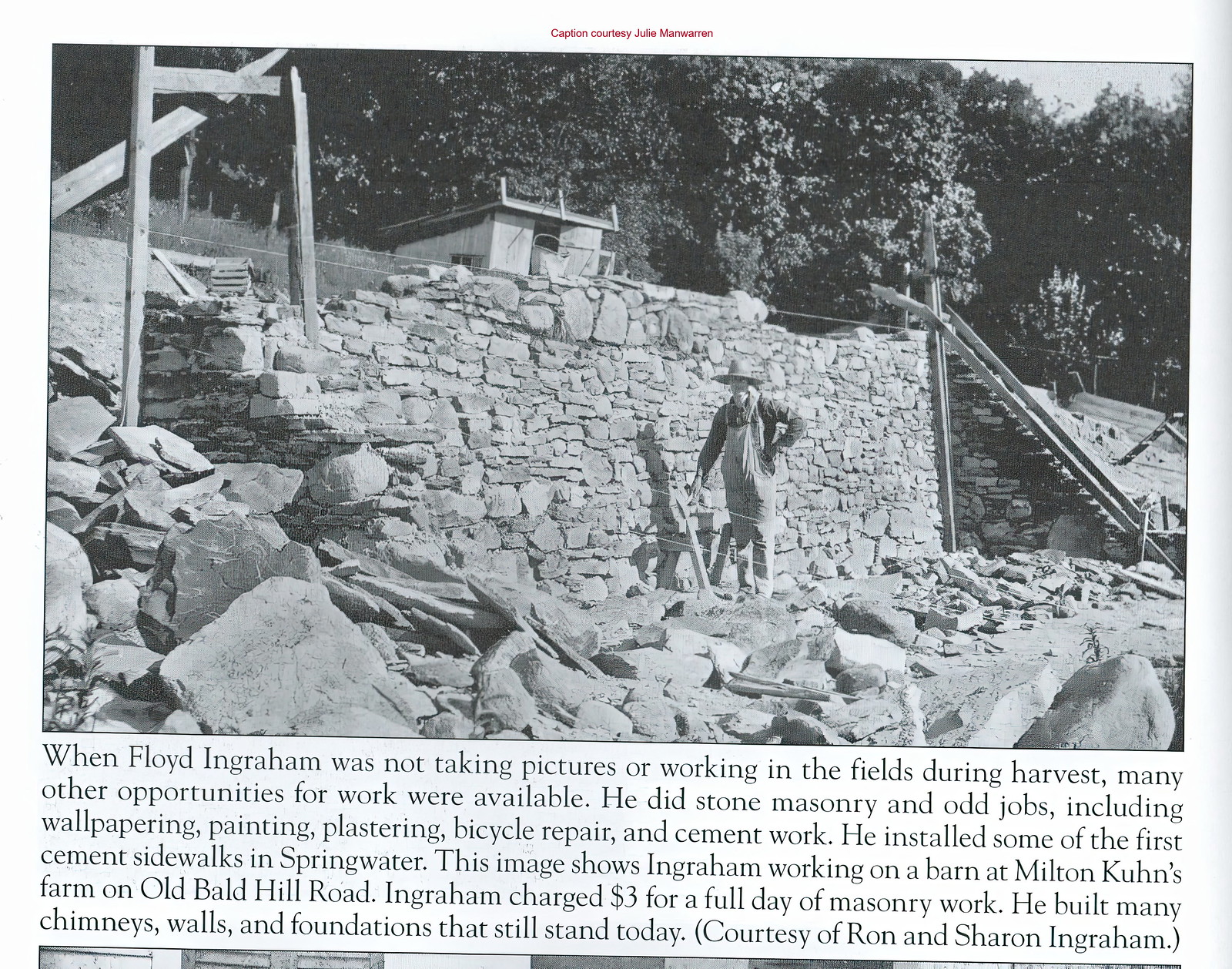The black and white photograph captures a farmer, dressed in overalls and a straw hat, working on a barn at Milton Coons Farm on Old Bald Hill Road. The image, which features a large stone wall taller than the man himself, shows him standing confidently with his left hand on his hip and his right hand resting on some tools. The farmer, possibly smiling, is Floyd Ingram, known for his diverse skills beyond farming, such as stone masonry, wallpapering, painting, plastering, bicycle repair, and cement work. Notably, Ingram installed some of Springwater's first cement sidewalks and built numerous chimneys, walls, and foundations that remain to this day. The caption, contributed by Julia Mann-Warren, appears in red at the top of the white-bordered image, while the detailed passage below the photo reads, "When Floyd Ingram was not taking pictures or working in the fields during harvest, many other opportunities for work were available. He charged $3 for a full day of masonry work." The passage also acknowledges Ron and Sharon Ingram’s contribution.